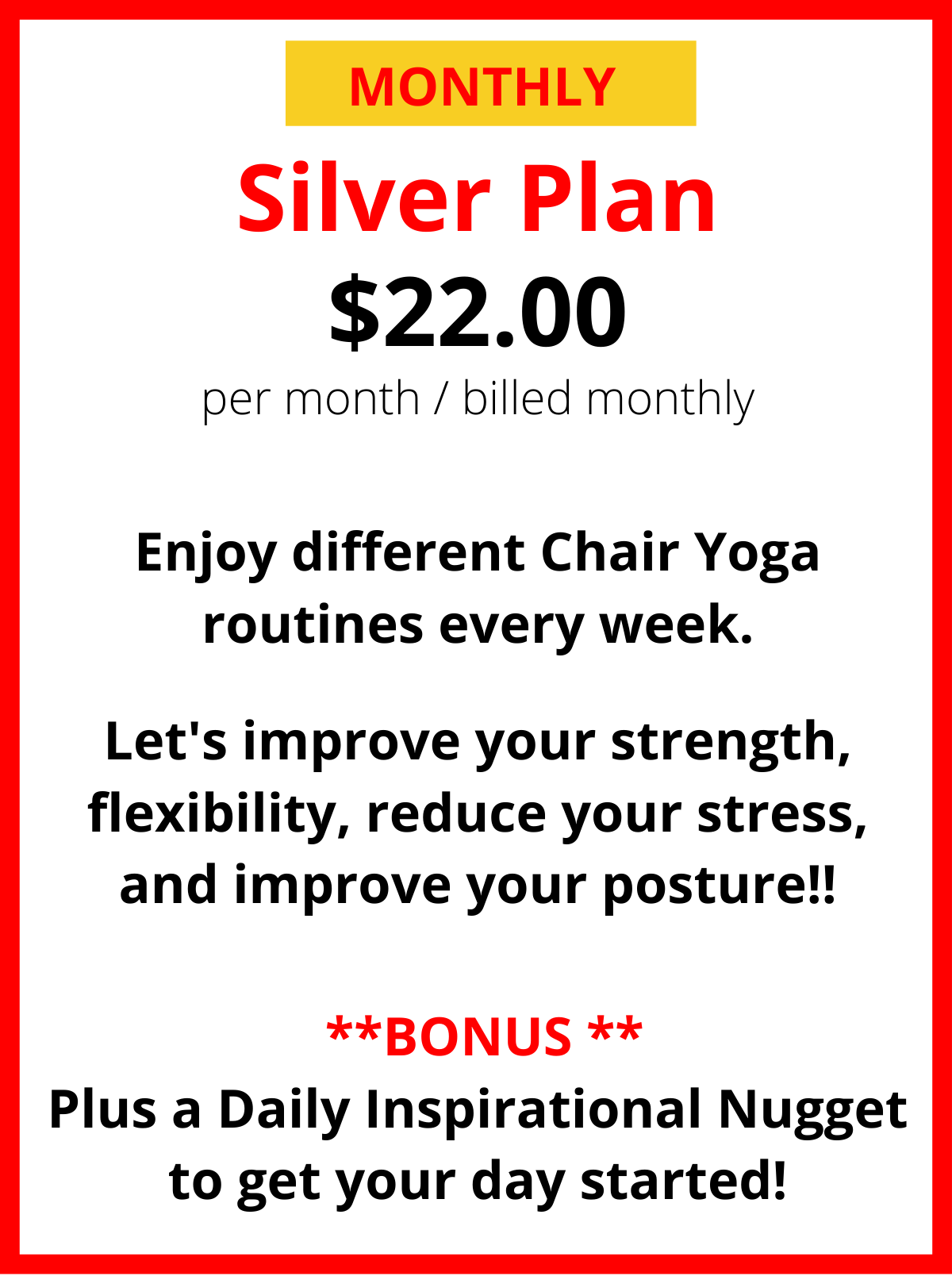A polished and detailed descriptive caption for the image:

---

This appears to be a promotional poster for a monthly subscription plan, likely displayed on a webpage. The design features a clean white background framed by a bold, red border. At the top of the poster, a gold, or perhaps mustard gold, rectangular banner contains the word "MONTHLY" in all caps.

Below the banner, the subscription type "SILVER PLAN" is prominently displayed in red uppercase letters, matching the red of the border. The cost is indicated in bold black text: "$22." Directly underneath, in non-bolded letters, it explains that this price is "per month, billed monthly."

Following this, a centered paragraph highlights the benefits of the plan:
"Enjoy different yoga routines every week. Improve your strength, flexibility, reduce your stress, and improve your posture!" This text is bold and ends with exclamation points.

A small separation follows, flanked by two asterisks on each side in red. The word "BONUS" in all caps introduces an additional perk: "Plus a daily inspirational nugget to get your day started," written in black.

The poster concludes with an invitation to sign up for this yoga plan, emphasizing the cost: "$22 a month."

---